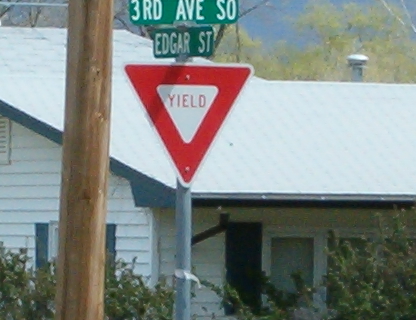A close-up photograph captures a yield sign mounted on a silver pole. The yield sign, characterized by its upside-down triangular shape, features a bold red background with a thin white border. Centrally placed within the red triangle is a smaller white upside-down triangle, inscribed with the word "YIELD" in prominent red letters. Above this sign, two green street signs are affixed to the pole. The top street sign, positioned horizontally with its left edge facing left and right edge facing right, reads "Third Avenue South." Directly beneath it, the second street sign is visible and labeled "Edgar Street."

In the background, a steeply angled roof of a white house is noticeable, adorned with blue shutters on both the front and sides. The bottom portion of the photo reveals the tops of thick, lush bushes, adding a touch of greenery to the scene. The overall composition highlights the yield sign while providing context through the visible street signs and elements of the surrounding environment.